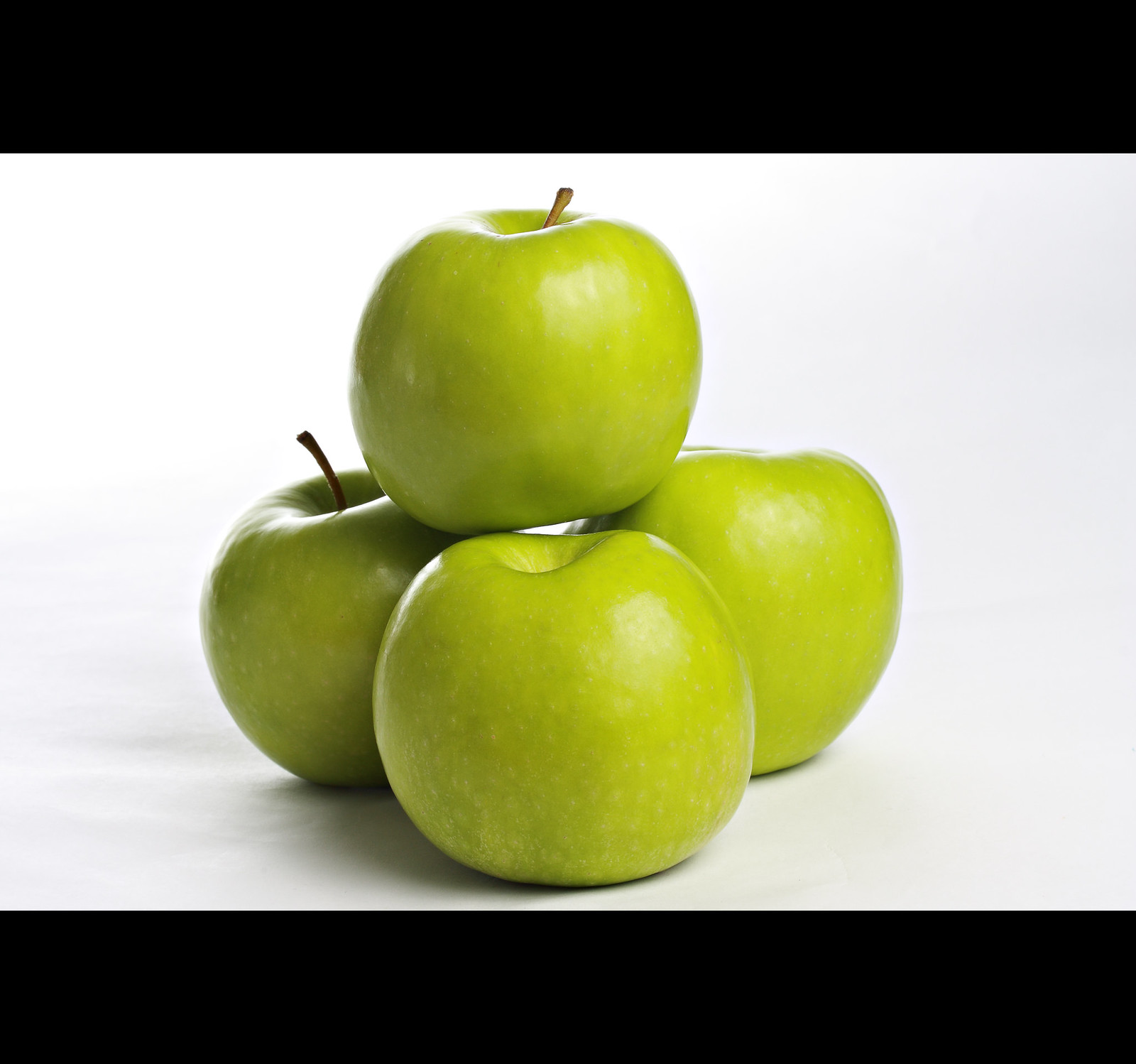The image is a professional photograph of four light green apples arranged in an aesthetically pleasing manner. Three of the apples are placed closely together in a triangular formation, with the fourth apple artistically perched on top of them. The apples appear flawless, shiny, and delicious, exhibiting a smooth surface with a couple of them retaining their stems. Positioned on a white cloth that covers a table, the setup introduces a slight texture with small wrinkles and shadows. The background features a minimalistic black and white frame, emphasizing the vibrant green hue of the apples. The natural light reflecting off the apples adds a luminous quality, highlighting their untouched, pristine condition.